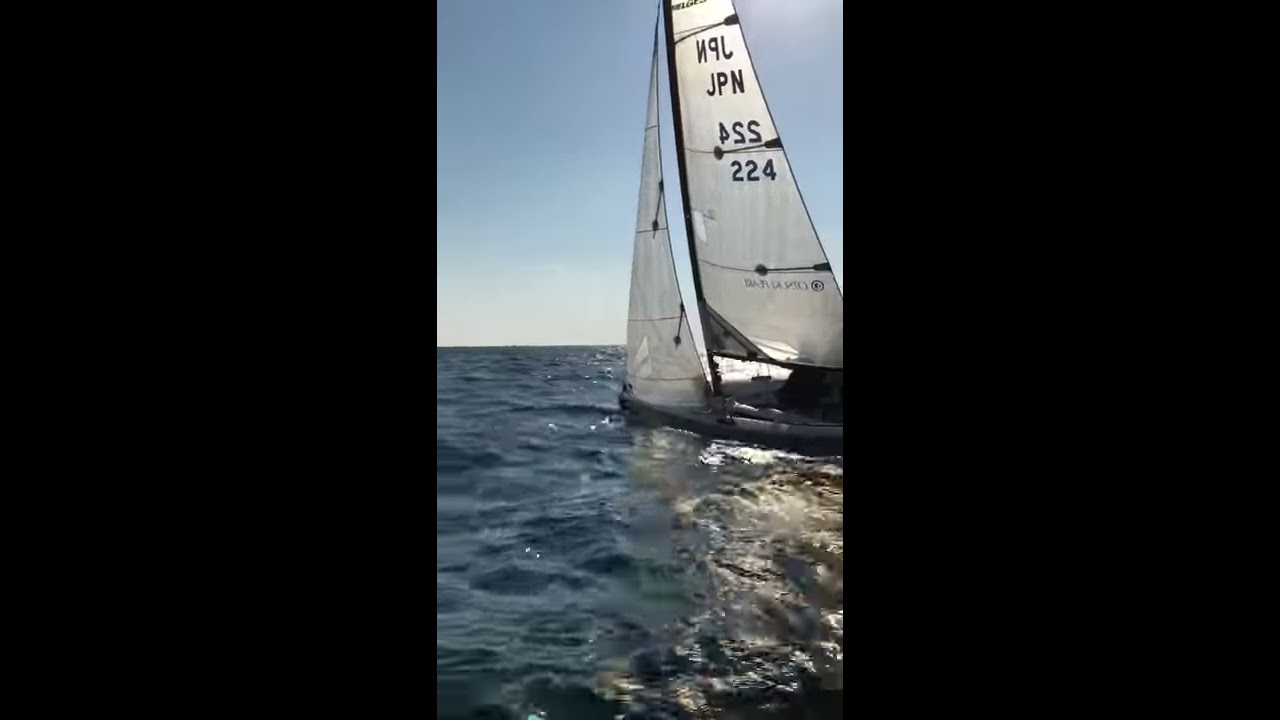The image is a vertically aligned rectangular photograph with thick black borders on either side, creating a narrow vertical rectangle that frames the main subject in the center. The lower half of the frame captures the ocean, which has a dark bluish-gray hue and appears somewhat rough with significant ripples, indicating choppy waters. Towards the right side of the image, a small sailboat with white sails is visible. The sails display black letters and numbers: "JPN" and "224." These inscriptions appear both normally and reversed in different sections of the sails. The sailboat has a dark blue body and is positioned partly in the middle, leaning slightly to the right. The upper half of the photo showcases a clear, light blue sky, which transitions to a slightly whitish hue near the horizon, suggesting the presence of distant clouds. The overall lighting suggests that the sun is behind the scene, casting a bright light on the sky while giving the ocean a darker, more shadowed appearance.